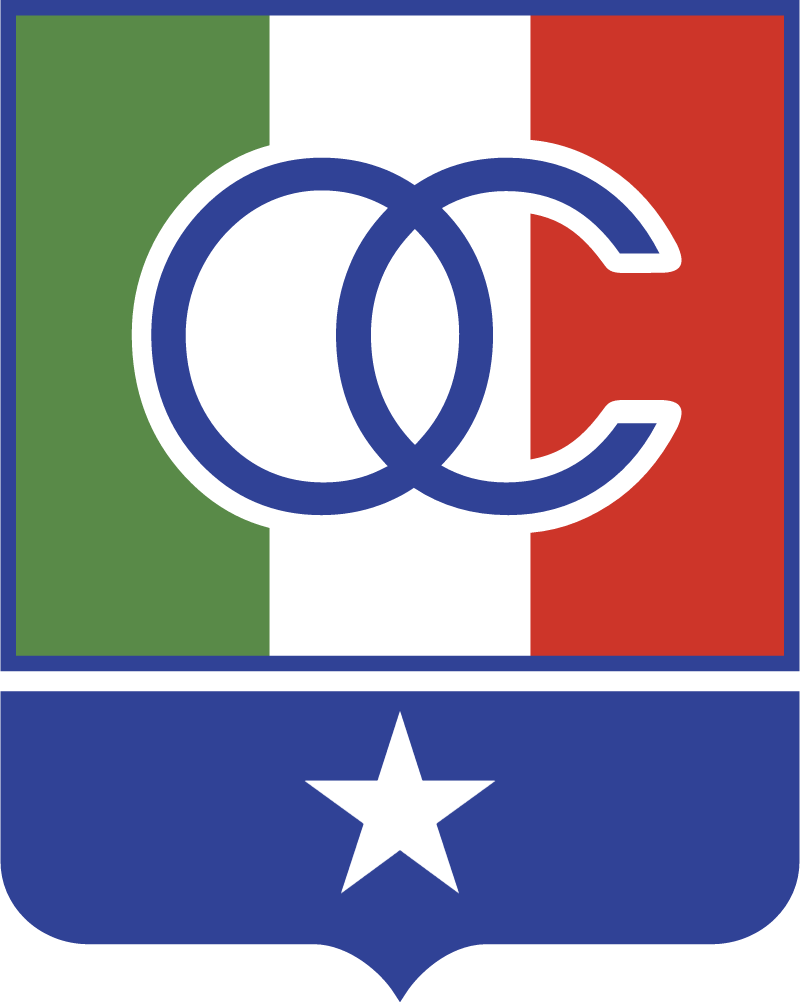This image depicts a distinctive shield-like logo, characterized by a blend of geometric designs and flag elements. The top portion of the logo is a rectangular block bordered in blue, divided into three vertical stripes reminiscent of a flag: green on the left, white in the middle, and red on the right, likely alluding to the Italian flag. Prominently centered atop these stripes are the blue interlaced letters 'O' and 'C,' designed in a manner that creates the visual effect of a Venn diagram, with the 'C' formed by leaving the right side open. These letters are outlined in white to ensure clarity against the flag's colors. Beneath this, the logo transitions into a blue, downward-pointing shape, curved at its sides and culminating in a point at the center. This portion is accompanied by a five-sided white star centrally positioned. The overall design combines traditional elements with modern visual coherence, resulting in a formal yet dynamic emblem.